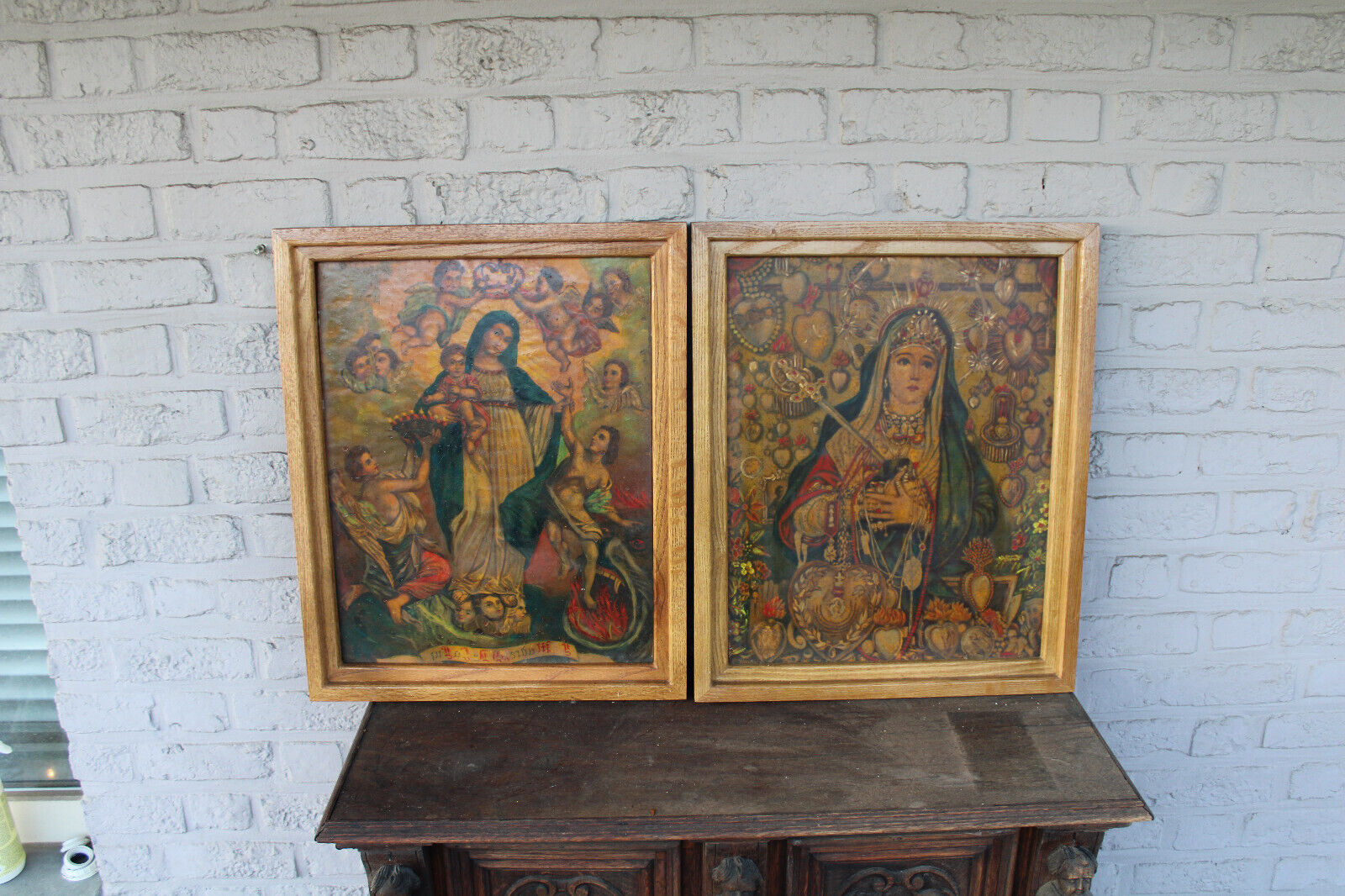This photograph captures two side-by-side, vertically-oriented Renaissance-style portraits encased in mid to light brown wooden frames. They rest on an old, dusty brown wooden table, positioned against a white painted brick wall. The ambience is accentuated by a glimpse of a window with blinds in the photo's left corner, hinting that the scene is outdoors.

The left portrait, known as "Mary Queen of Angels," vividly depicts Mary draped in a blue veil and wearing a brown belt over her flowing dress. She tenderly cradles baby Jesus in her right arm. Surrounding Mary are cherubs; some are flying above her head, possibly carrying a crown, while others are seen in the foreground, along with a group of children and adults reaching up to her. A subtle sun-like glow can be seen behind her. The painting is imbued with fine details and a soft, faded color palette dominated by darker reds and greens.

The right portrait is labeled "The Immaculate Heart of Mary." In this depiction, Mary dons a dark taupe veil that originates from a crown atop her head and cascades down her shoulders. Her serene and pious expression complements the intricate background adorned with hearts, plants, and flowers. This painting shares the Renaissance-era aesthetic with its lush, detailed motifs and a similar muted color scheme.

Below both portraits, the brown wooden table appears worn and is pushed firmly against the wall, adding to the vintage atmosphere of the photograph.